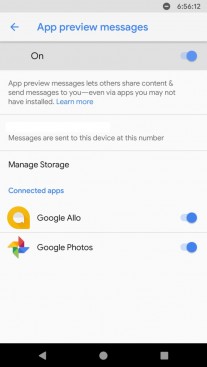This image depicts a webpage dedicated to "App Preview Messages." The heading "App Preview Messages" is prominently displayed in blue at the top left corner, accompanied by a left-facing arrow. The feature is currently enabled, indicated by an "On" label and a fully blue slider. The page explains that "App Preview Messages" allows others to share content and send messages to the user, even through apps that may not be installed on the device, with a "Learn More" link in blue for additional information. It also informs the user that messages will be sent to the current device and associated number.

Below this, there are options to manage storage and connect apps. The first app shown is Google Allo, displayed with a yellow balloon icon featuring a white center. This app is turned on, also highlighted by a blue indicator. The second app is Google Photos, represented by an icon with red, yellow, green, and blue leaves intertwined, accompanied by the label "Google Photos" in blue text.

The bottom of the webpage features a black strip containing three navigation symbols: an arrow, a circle, and a box, located on the right side.